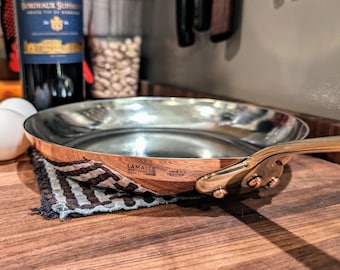This detailed photograph captures a pristine copper-clad frying pan with a stainless steel interior, approximately 12 inches in diameter, positioned on a light brown wooden table. The copper handle extends slightly forward and to the right. Beneath the pan is a white cloth with vertical black stripes, folded neatly. To the left of the pan, near the edge of the table, lie two white eggs. Just above the eggs, there is a black bottle with a blue label, its text indistinct. Beside the bottle sits a container fully filled with peanuts. The backdrop on the right side of the image features a simple gray wall, devoid of any other objects, emphasizing the scene's focus on the cooking elements. The overall composition suggests a clean, well-maintained kitchen setting, possibly preparing for a meal.